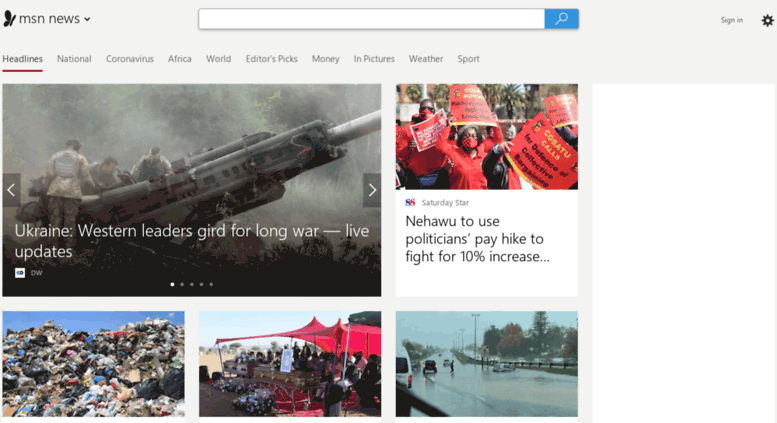The image is a screenshot of an MSN News webpage, capturing a variety of headlines and sections. At the top of the page, the navigation bar lists different categories such as National, Coronavirus, Africa, World, Editor's Picks, Money, In Pictures, Weather, and Sport. Below the navigation, the main headline reads "Ukraine: Western Leaders Brace for Long-Haul," with supplementary stories including a live update on the situation and a piece on using politicians' recent pay hikes to argue for a 10% increase.

The webpage features several smaller images that accompany the news stories: 
1. Protesters holding signs.
2. A torrential rainstorm affecting a busy road.
3. A significant accumulation of trash indicating an issue with waste management.
4. A solemn burial ceremony with two coffins visible, suggesting a communal mourning.

At the top right corner of the page, options to 'Sign In' and icons for 'Get' and 'Settings' are displayed, offering users quick access to personal accounts and customization features.